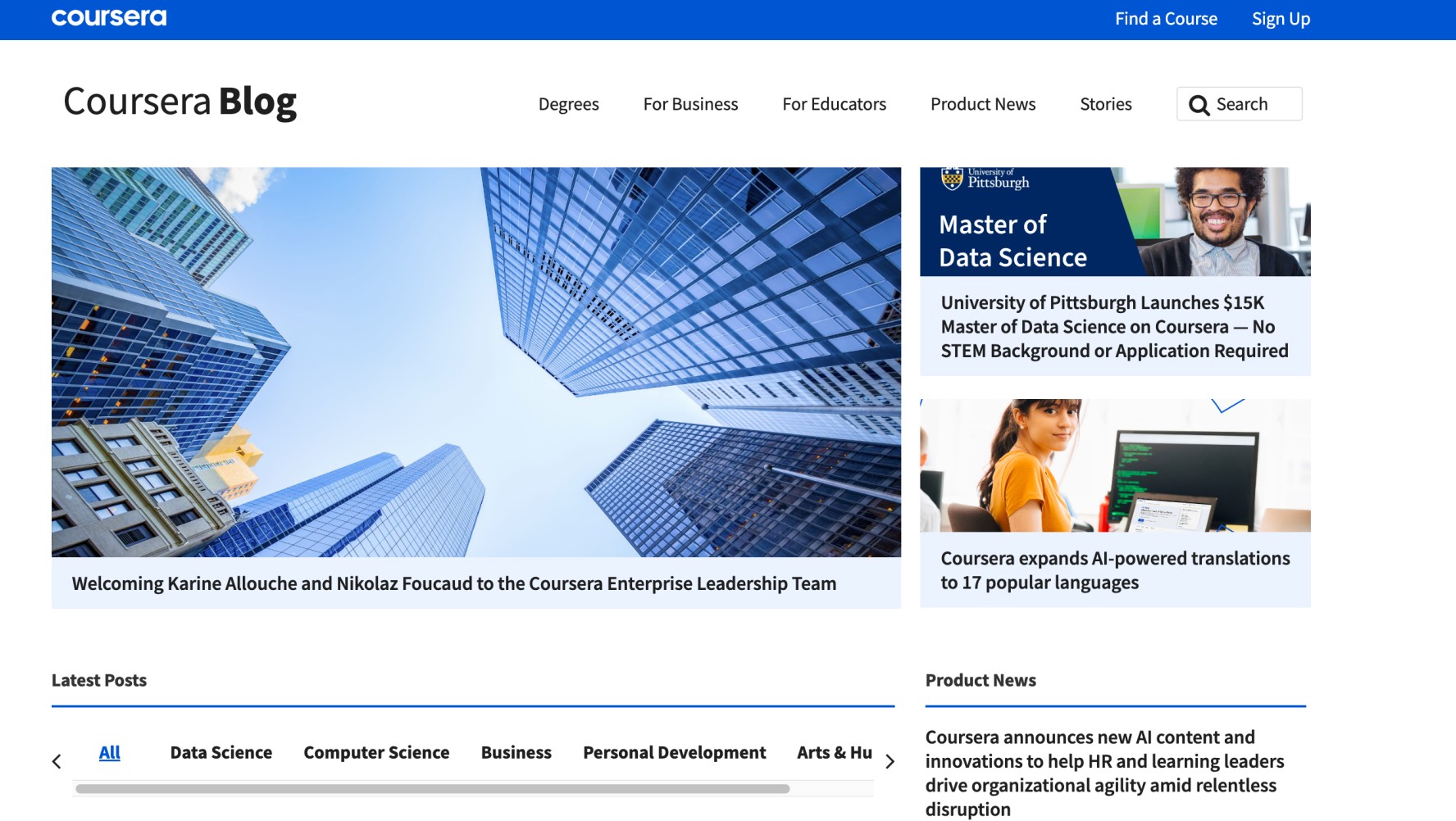The web page features a prominent horizontal bright blue banner running from left to right. On the left side of this banner, the word "Coursera" is displayed in all lowercase white letters. On the right side, in smaller white font, the phrases "find a course" and "sign up" are visible. Below this header area, "Coursera" is written in larger black font, with "blog" in bold black lettering next to it.

A series of menu headings extends from just left of center to the right side, including "Degrees," "For Business," "For Educators," "Product News," "Stories," and "Search."

Dominating the main content area beneath the banner, there is a horizontal image depicting a view of skyscrapers from below, giving the impression of looking upwards from the ground.

Directly beneath the image, a headline states, "Welcoming Corinne Alouche and Nicholas Foucaud to the Coursera Enterprise Leadership Team."

At the very bottom, a section titled "Latest Posts" highlights topics such as "Data Science," "Computer Science," "Business," "Personal Development," and "Arts," with the word "All" in turquoise and an arrow indicating the ability to scroll for more content.

On the right side of the page, there is a vertical section with two horizontal images, seemingly advertisements. The first ad, under a blue area labeled "Pittsburgh," displays a title in white font, "Master of Data Science." To the right, an image of a man with glasses, a beard, and a mustache wearing a jacket and nice shirt is shown. Under this, black font reads, "University of Pittsburgh launches 15K Master of Data Science on Coursera - no STEM background or application required."

The second ad features an image of a woman looking at the viewer while facing a computer screen with green text. This ad announces, "Coursera expands AI-powered translations to 17 popular languages." 

At the bottom of the vertical section, under the heading "Product News," a horizontal blue line is followed by a new announcement: "Coursera announces new AI content and innovations to help HR and learning leaders drive organizational agility amid relentless disruption."

This detailed description captures the layout and specific content of the web page in a structured and comprehensive manner.